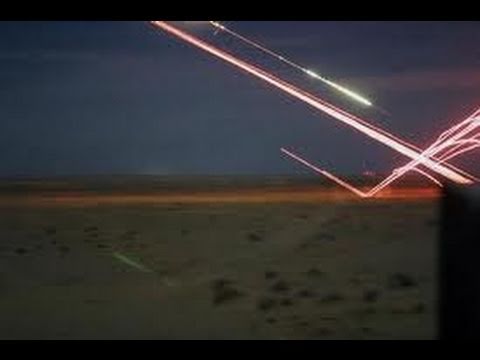This very blurry nighttime photograph appears to be a desert landscape with a horizon line roughly at the midpoint of the image. The sky, partially cloudy, forms the backdrop against which streaks of light are vividly noticeable. These streaks, predominantly orangish-red and originating mainly in the top right quadrant, seem to descend and sometimes ricochet off the sandy ground. Among them, there is a particularly distinctive and bright yellow streak, while hints of white and green are also visible in one of the light trails. Although the resolution is low, the overall impression is that of mysterious luminous phenomena, potentially resembling fireworks, illuminating the night desert scene.